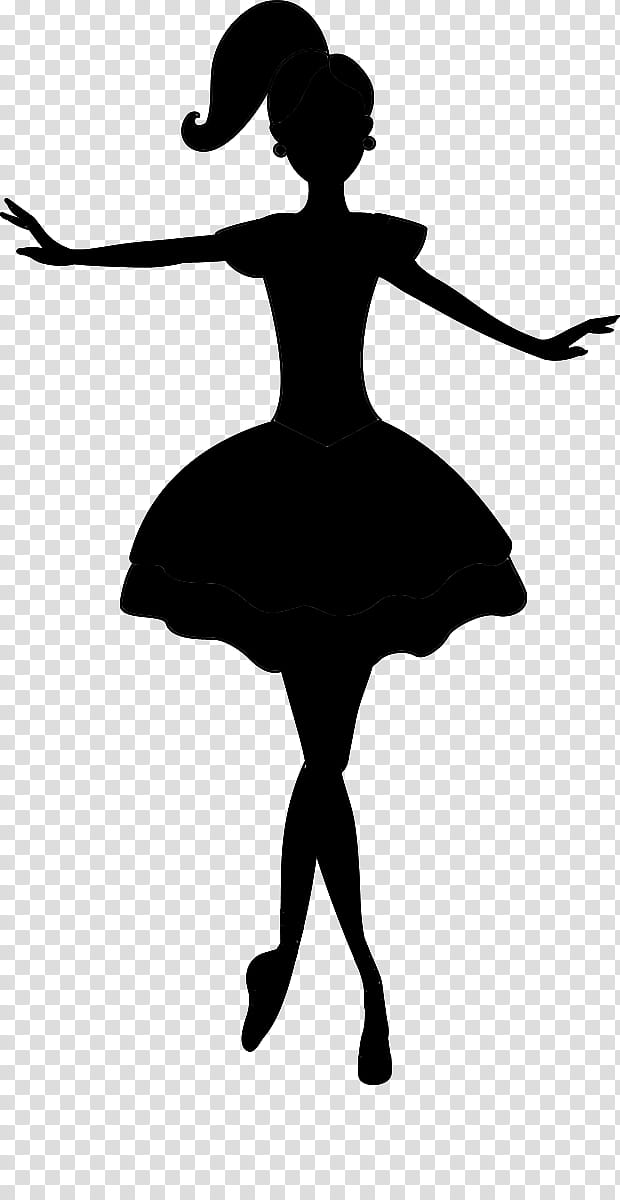This image is a piece of digital art in the form of a PNG file. The background is a gray and white checker pattern, typical of images meant to have transparent backgrounds. Featured prominently in the center is the black silhouette of a cartoonish ballerina. The ballerina, depicted from the front, has a high ponytail that extends to the left side of her head. Her figure includes large circular earrings and a short-sleeved dress that resembles a tutu with subtle wavy details. She stands on her tippy toes with her legs crossed, arms extended elegantly to the sides. The overall appearance strongly suggests the classic caricature of a ballerina, akin to a Barbie-like figure with exaggerated features typical of vinyl stickers or clip art.